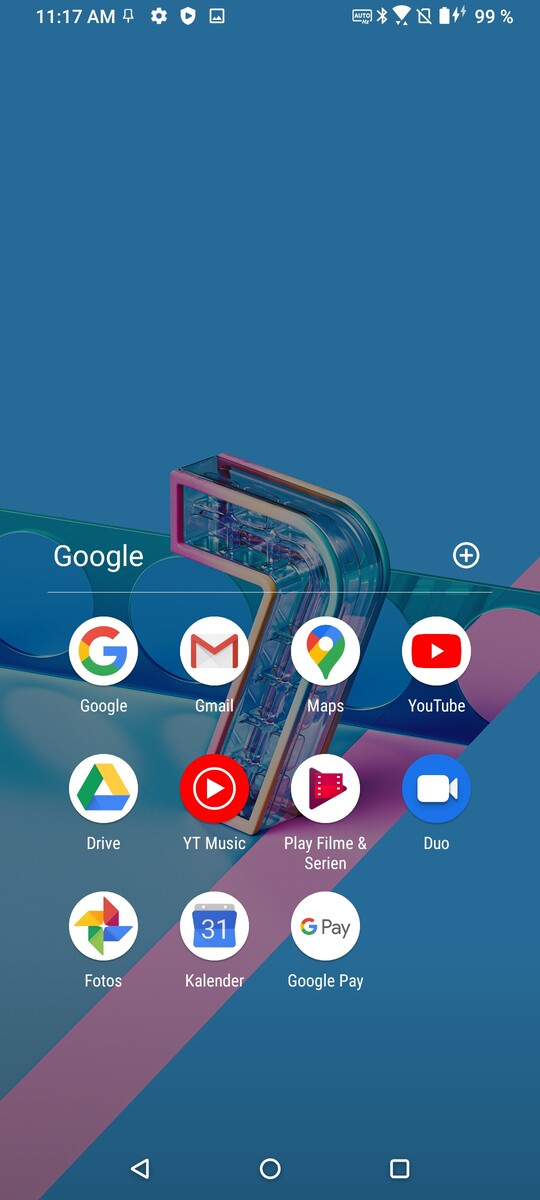The image showcases the home screen of a Google smartphone. At the top of the screen, the clock displays the time as 11:17 AM. Various status indicators are visible, including the settings cogwheel, Bluetooth connectivity enabled, and a battery life at 99%. The wallpaper features a modernistic logo with the number "7" stylized as a sideways "V." This design comprises a pink strip alongside a piece of metal with perforations, overlaid with a three-dimensional number "7" highlighted along its edges.

Below this striking backdrop, a row of app icons occupies the screen. These are predominantly Google-owned applications such as Google Chrome, Gmail, Maps, YouTube, Drive, YouTube Music, Photos, and Google Pay, solidifying the identity of the device as a Google smartphone. The arrangement and choice of apps emphasize its extensive integration with Google's ecosystem.